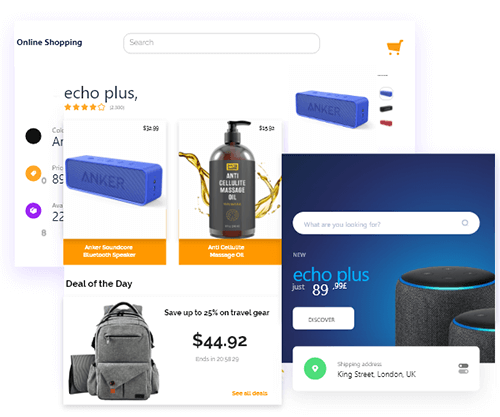The image displays a shopping website divided into three distinct panels. 

### Top Panel:
- **Background**: White
- **Text**: "Online Shopping" in black print with capitalized 'O' and 'S'
- **Features**:
  - **Search Bar**: Grey text placeholder
  - **Shopping Cart Icon**: Highlighted in orange, located on the right side

### Middle Panel:
- **Product 1**: Echo Plus
  - **Rating**: Four stars
  - **Review Count**: Displayed next to the rating
  - **Color Options**: Three small circles representing different colors
    - Black
    - Orange
    - Purple
    
- **Product 2**: Anker Bluetooth Speaker 
  - **Text**: "Anker" in top-left corner
  - **Description**: Bluetooth Speaker
  - **Color Options**:
    - Blue (circled)
    - Black
    - Red

### Bottom Panel:
- **Pop-Up Window**: Displays three different products under the Echo Plus section
  - **Top Left**: Anker Bluetooth Speaker
  - **Middle**: Anti-Cellulite Massage Oil
  - **Bottom**: Deal of the day—save up to 25% on travel gear
    - Listed Price: £44.92
    - Countdown Timer: 20:58:29
    - Additional Info: "See all deals"
    - Featured Image: Backpack

### Additional Features:
- **Pop-Up Info**:
  - **Price**: Echo Plus listed at £89.99 (displayed in British pounds)
  - **Shipping Banner**: White banner with green circle containing a map icon. Text reads "Shipping Address: King Street, London, UK."

This detailed description captures the layout and key details of the shopping website image.